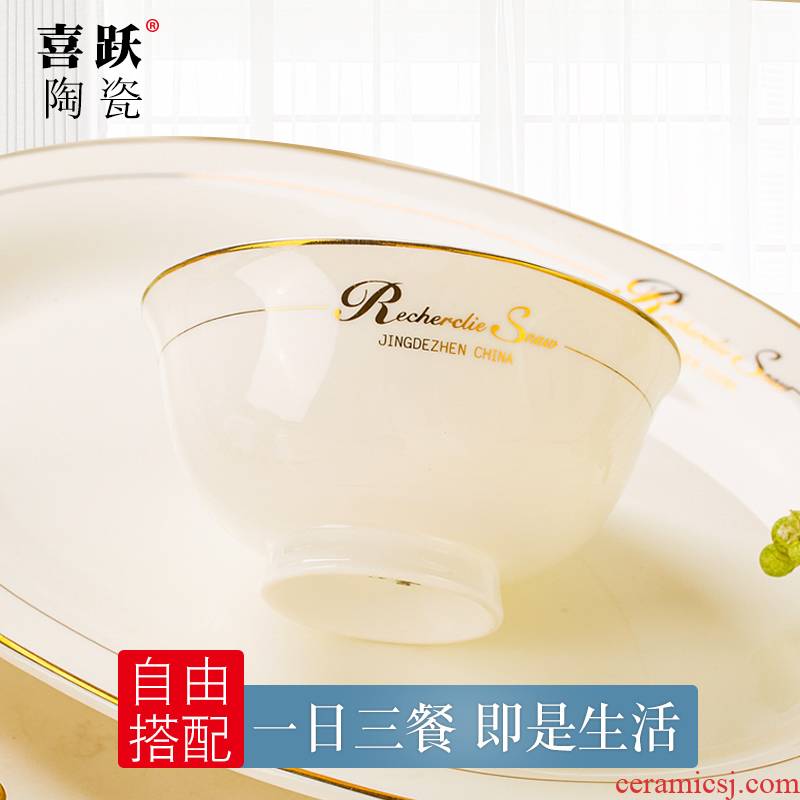The image depicts a detailed layout of fine porcelain china, consisting of an oval-shaped platter and a smaller, circular bowl. Both pieces are adorned with delicate gold trim, with the bowl featuring an additional gold stripe beneath the rim. The bowl displays cursive text that appears to read "Resherkly," followed by indistinguishable characters, and below this, "Jingdezhen, China" is clearly marked. In the upper left corner, there are four Chinese characters next to a registered trademark symbol. At the bottom left of the image, a red square containing white Chinese characters is adjacent to a blue horizontal rectangle with further Chinese script. The background is a pristine white, and the entire image has a golden hue. In the lower left-hand corner, the URL "CeramicSJ.com" is visible.